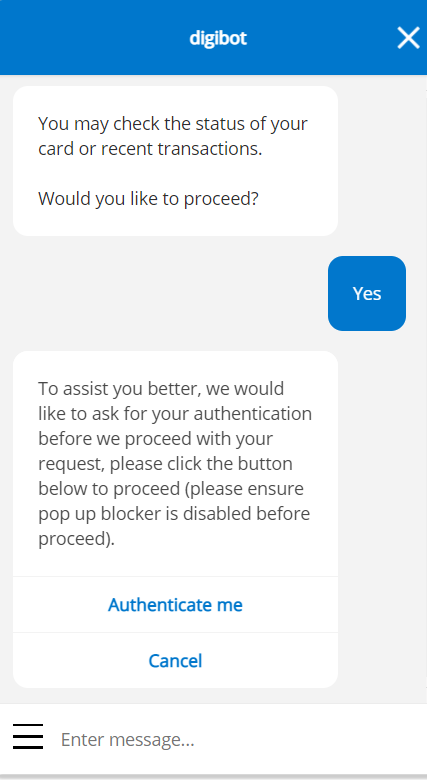**Caption:**

The image displays a digital interface with specific sections and instructions. At the top, a blue bar spans across the screen, featuring the word "Digibot" in white, centered, with a white "X" on the right-hand side. Below, on a gray background, a white box with black text on the upper left reads: "You may check the status of your card or recent transactions. Would you like to proceed?" To the right of this message, a blue box contains the word "Yes" in white text.

Further down on the left-hand side, another message in matching formatting states: "To assist you better, we would like to ask for your authentication before we proceed with your request. Please click the button below to proceed. Please ensure pop-up blocker is disabled before proceed." Below this, a blue button in the center reads "Authenticate me" with a "Cancel" option underneath.

At the bottom left, three black horizontal bars are visible next to a gray area designated for entering another message. The interface aims to guide users through checking their card status and transaction history while ensuring proper steps are taken for authentication.